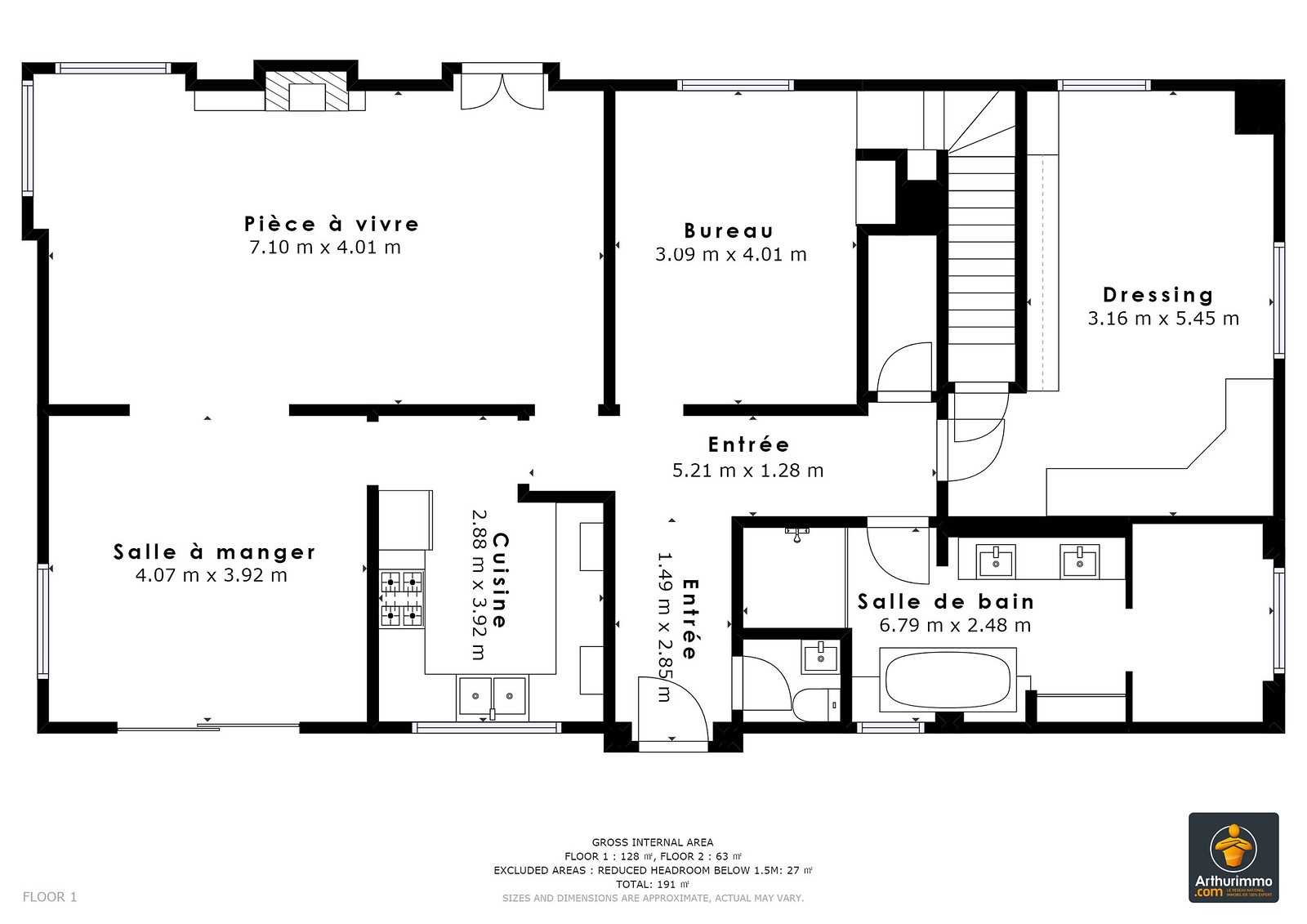**Descriptive Caption:**

The image is a detailed black-and-white blueprint of a home. On the upper left-hand side, there is a room labeled "Piche de Verve" measuring 7.10 meters by 4.01 meters. This room features a window in the upper right-hand corner and a fireplace in the bottom left-hand corner. Adjacent to this room is the "Salet de Manager," a dining room measuring 4.0 meters by 3.92 meters. To the right of the dining room is the kitchen, labeled "Cuisine," which measures 2.88 meters by 3.92 meters. Next to the kitchen is the "Entrée," or entrance, measuring 1.49 meters by 2.85 meters.

From the entrance, a hallway, also labeled as "Entrée," extends to the right, measuring 5.21 meters by 1.28 meters. Positioned north of this hallway is the office, or "Bureau," which measures 3.09 meters by 4.01 meters. Adjacent to the office is a dead-end hallway, with a staircase leading upwards.

South of the hallway is a bathroom, labeled "Salet de Bain," which measures 6.79 meters by 2.48 meters. This bathroom contains a bathtub positioned in the southern part of the room as well as two sinks. To the right of the bathroom is an empty room, and directly north of that, separated by a wall, is a dressing room measuring 3.16 meters by 0.545 meters. The blueprint appears to be created by Elunio.com and is labeled as floor plan number one, with some areas excluded and a total internal floor area of 1.91 meters by 1.